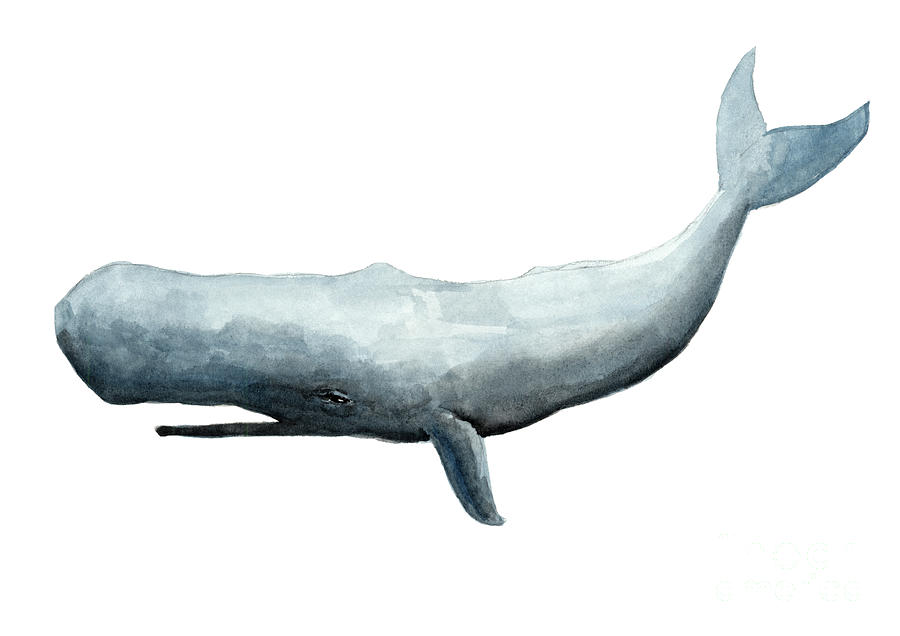The image is a painting of a whale, specifically showcasing the left side of the animal, set against a completely white background devoid of any water or other elements. The whale, depicted with a combination of blue and gray hues, has a distinctly large nose and mouth, the latter partially open revealing rows of teeth. Its eye, marked with a black pupil and a small white dot, exudes a sense of illness or distress. The whale features a dark blue belly which gradually transitions to a lighter blue toward the top, contributing to a sense of depth in its portrayal. It has a single visible fin hanging down on its left side and a tail raised behind it consisting of two fins, though only the left one is visible. The painting lacks intricate textures, giving it a somewhat sketch-like appearance, and the whale's jagged outline enhances its rough, simplistic style. No signature is present to identify the artist. The overall mood suggests the whale is in need of help, accentuated by the somber look in its eyes.